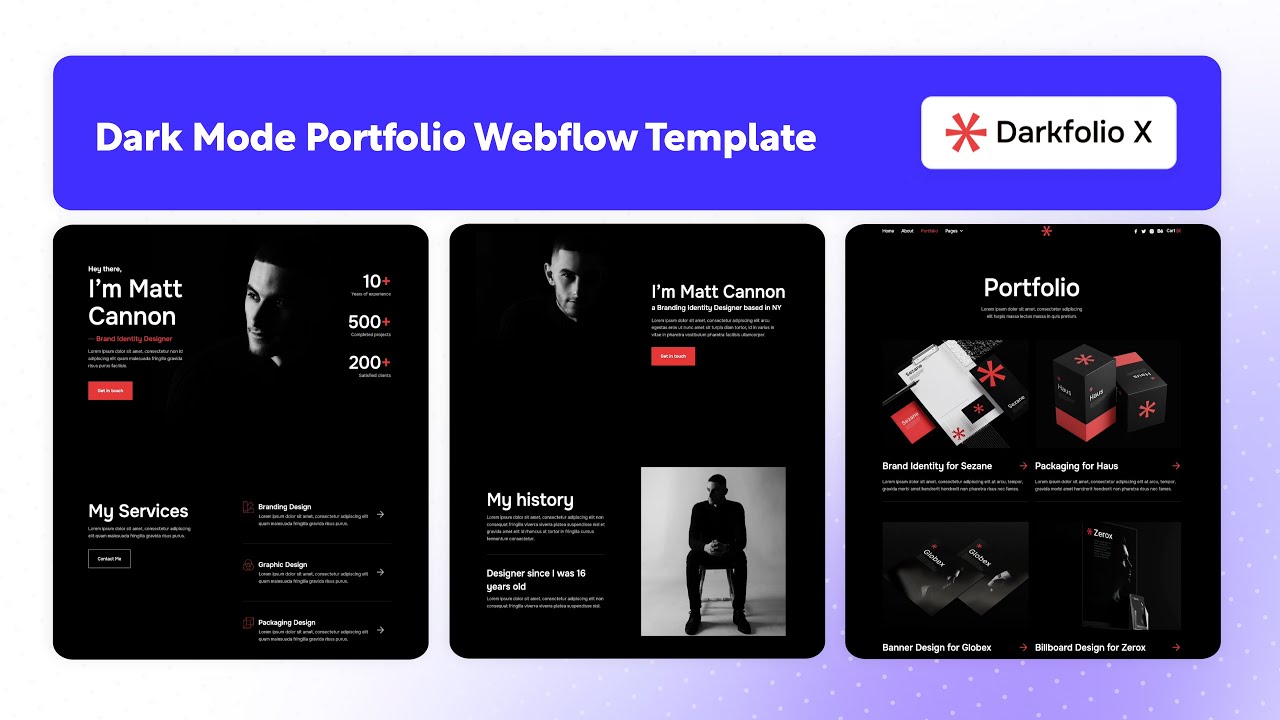The up-close image appears to be an advertisement for a company called Dark Folio X. The top section features a bright blue bar with white text that reads, "Dark Mode Portfolio Webflow Template," and in the top right corner there's a white box that says "Dark Folio X" with a red asterisk to the left of "Dark Folio."

Below this, the image is divided into three vertical, rectangular sections with a black background and white text. 

- The left section prominently displays the text, "Hey there, I'm Matt Cannon," alongside a shadowy picture of what is presumably Matt Cannon's face. It also includes a caption that says "My Services," detailing his expertise in branding design, graphic design, and packaging design.
  
- The middle section also states, "I'm Matt Cannon," and includes the subtitle "My History," describing his background and history in design since the age of 16. 
  
- The right section is labeled "Portfolio" and lists examples of his work, including "Brand identity for Suzanne," "Packaging for Haas," "Banner design for Globex," and "Billboard design for Xerox."

Each section features a mix of white text with some red accents against a black background. There are small images within the sections, including side views of his face and a picture of him sitting on a chair, but these are not very clear. The overall design uses a minimalist color scheme of blue, black, white, and red.